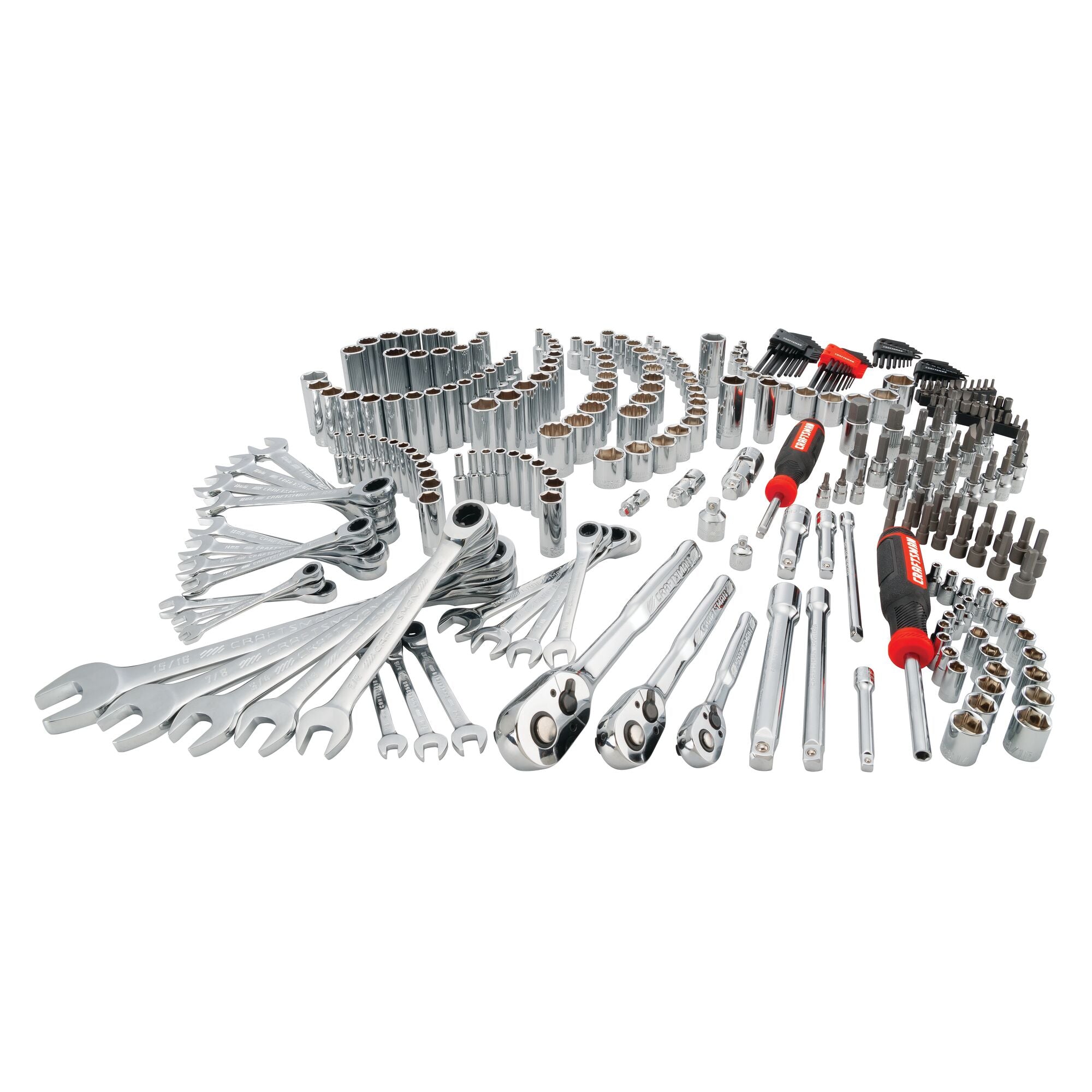The photograph showcases an extensive tool set meticulously laid out on a white background. The set features an array of metal ratchets and wrenches of varying sizes, organized in rows and by size. Prominently, there are a few black and red-handled screwdrivers designed to accommodate different bits, with accompanying extensions to increase their length. Also included are numerous socket heads for the ratchets, arranged neatly in rows. In the background, sets of Allen wrenches are visible, encased in both black and red holders, with the ends of the wrenches protruding to show the various sizes. This comprehensive tool set is displayed in a way that highlights the variety and organization of each component, emphasizing its utility and design.